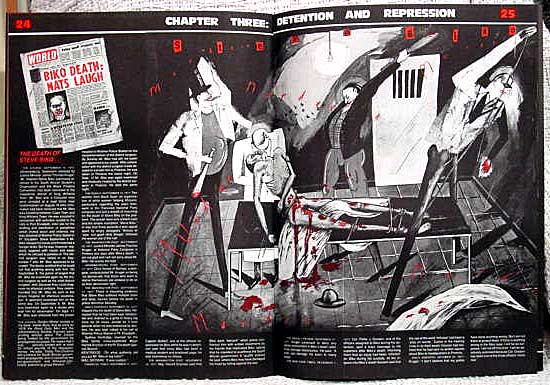This detailed black-and-white sketch, accentuated with stark red blood, appears on page 24 of a magazine or comic book. Titled "Chapter 3: Detention and Repression," the gripping scene unfolds in what seems to be a cell or an enclosed area. Two animated characters, one in a top hat and white jacket, the other sporting a long white beard, are positioned at the head and foot of a human victim lying on the floor. They wield swords and other instruments stained with blood, indicating an ongoing murder. Blood pools around the victim and splatters across the scene, heightening the sense of brutality. In the background, a third figure, potentially a detective or observer, holds a sword in his left hand, adding to the tense atmosphere. Overlooking the carnage, the upper left corner of the image features a newspaper clipping with the headline "Beko's Death, Nat's Laugh," from The World, enhancing the narrative's grim context. The bottom of the page features tiny, hard-to-read text, contributing to the article's depth. The subsequent page number, 25, is noted in the top right corner, promising more to this dark and intense storyline.